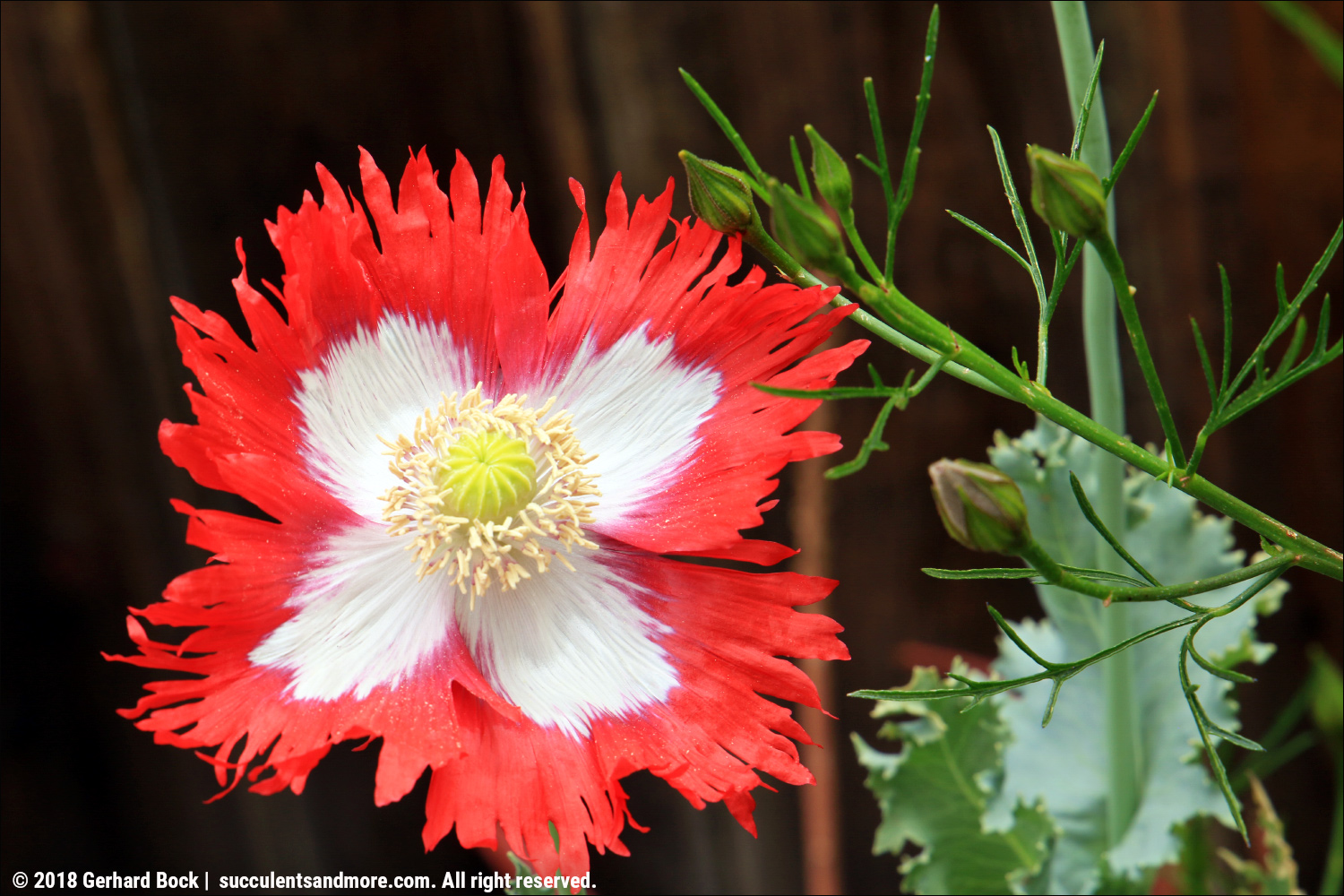Close-up photograph of a brightly colored flower with multiple wispy, sharp-edged petals. The tips of the petals are a fiery red, transitioning to white near the center. The flower features a green bulb with slightly greener tendrils extending toward the center. Around the edges of the bulb are small cylindrical yellow shapes. To the right of the flower, green vines and jagged-edged leaves are visible against a predominantly black background with hints of brown. There are additional buds and stems indicating the presence of more blooms in various stages of growth. At the bottom left-hand corner of the image, in white font, it reads: "© 2018 Gerhard Bach, succulentsandmore.com, All rights reserved."